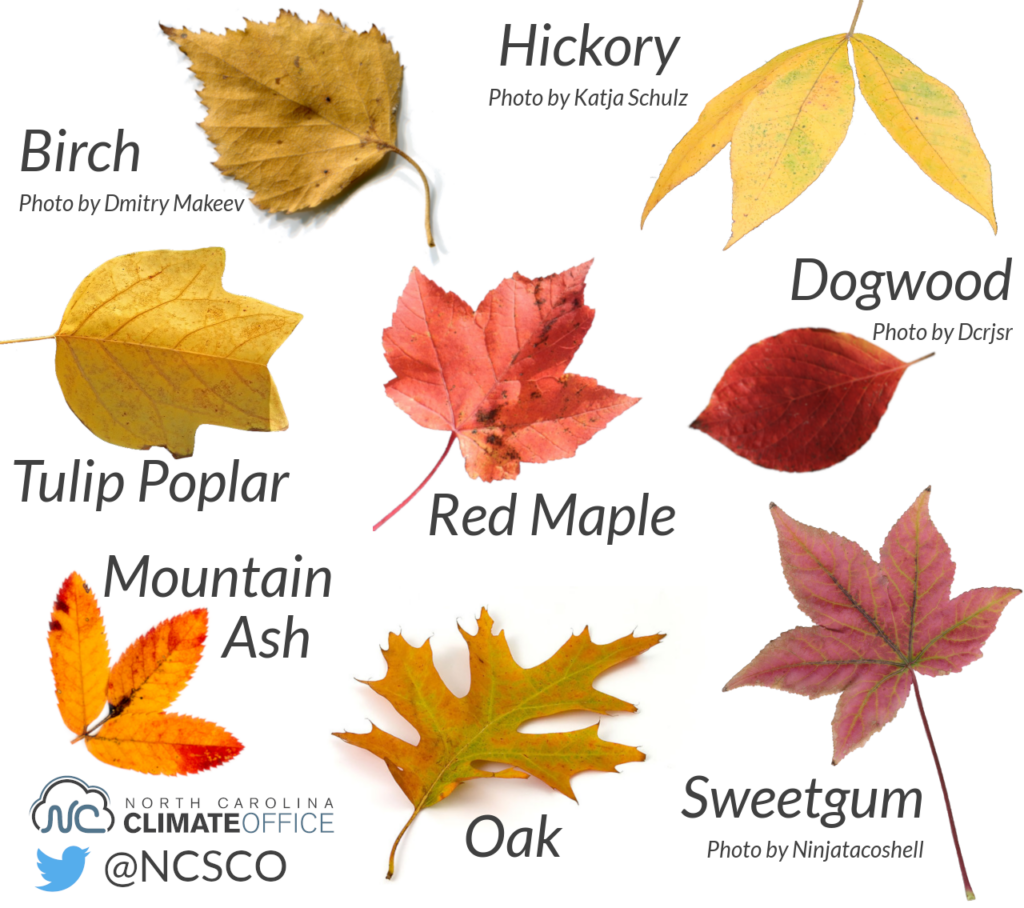This infographic features a detailed chart of eight different types of leaves arranged against a white background, showcasing their vibrant autumn colors. The chart includes yellow birch leaves photographed by Dimitri McKeeve, hickory leaves by Katja Schultz, and a tulip poplar leaf. A red dogwood leaf with a photo credit to DCRJSR, an orange mountain ash leaf, and a red leaf of the red maple are also included. Additionally, an oak leaf is depicted with a mixture of yellow, orange, and green hues, while the sweetgum leaf, photographed by Ninja Taco Shell, displays a brilliant red. At the bottom left corner, the emblem of the North Carolina Climate Office (NC) is situated next to the organization's Twitter handle, @NCSCO. Photo credits to Katcha Schultz, DCRJSR, and Ninja Taco Shell are noted underneath the respective leaves.